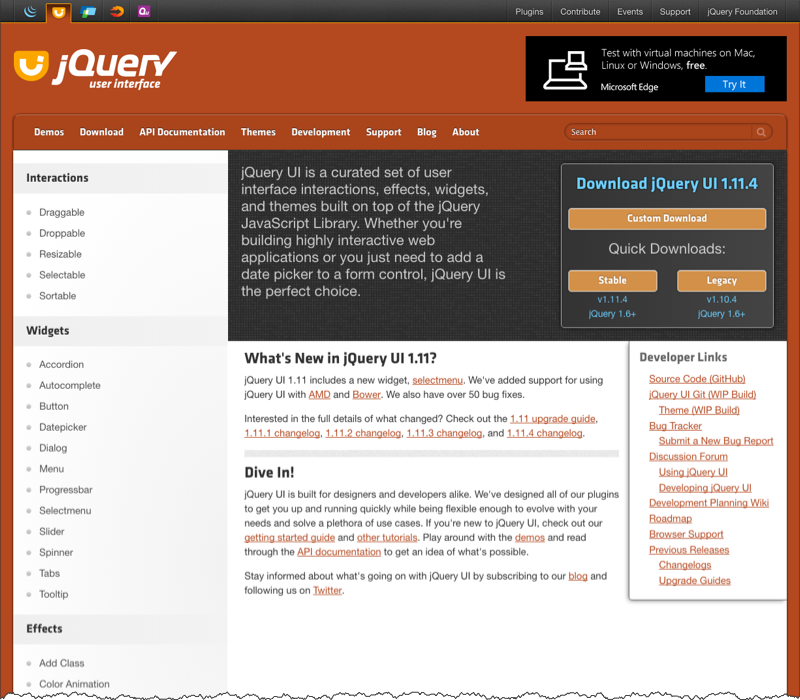The image is a detailed screenshot of a jQuery User Interface website. The bottom edge of the image features a thin, jagged line, resembling the appearance of a manually torn page. The website is framed with a rusty red border on both the left and right sides, and the same rusty red color forms a band across the top.

At the top of the page, there is a thin black bar containing various categories such as "Support" and several other unreadable options, along with five colorful icons situated on the top left corner whose specific details are not discernible.

The primary header of the website reads "jQuery User Interface," with "jQuery" appearing in white text against the rusty red background. Directly to the right of this header, there is a prominent black rectangle. Inside this rectangle is a blue "Try It" button, a white outline illustration of computers, and text that includes the words "Microsoft Edge" and "Test" among other unreadable elements.

The background beneath this section transitions to white. A column on the left side lists various categories: "Interactions," "Widgets," and "Effects." Under "Interactions," there are five options: "Draggable," "Droppable," "Resizable," "Selectable," and "Scalable." The "Widgets" category features twelve options, including items such as "Button" and "Accordion," although many are too small to read clearly. The "Effects" category contains a few options followed by the torn page effect at the bottom.

On the right side of the page, there is another black rectangle that reads "Download jQuery UI 1.11.4," suggesting it's a version number. Options for a "Custom Download" or "Quick Downloads" are provided. The text within this section explains, in white font on a black background, that "jQuery UI is a curated set of user interface interactions, effects, widgets, and themes built on top of the jQuery JavaScript library. Whether you're building highly interactive web applications or you just need to add a date picker to a form control, jQuery UI is the perfect choice."

The remainder of the page features a white background with black and red text. All the red text is clickable. There are numerous developer links on the right-hand side, a section detailing "What's New in This Version," and an invitation to "Dive In."